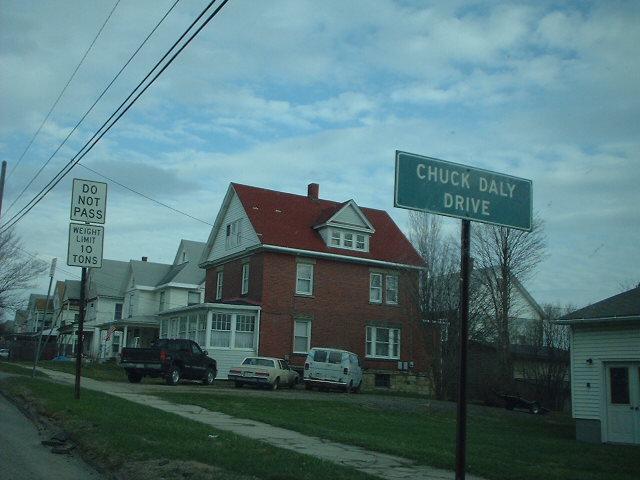This photo, taken from a vehicle on an overcast day, showcases a suburban residential street. The foreground features a green sign with white border and text on a metal pole reading "Chuck Daly Drive." Nearby, another pole supports a white, rectangular "Do Not Pass" sign with "Weight Limit 10 Tons" displayed beneath it. Both signs stand adjacent to a gray sidewalk and lush grass yards. The backdrop reveals a row of closely-knit houses, predominantly highlighted by a red brick two-story house with a white enclosed porch. Parked in front of this central house are three vehicles: a black pickup truck, a cream-colored sedan, and a white van. Surrounding it are additional white houses with gray roofs, under a sky that's light blue with gray clouds. Power lines stretch across the upper left corner, completing this detailed snapshot of a picturesque neighborhood.